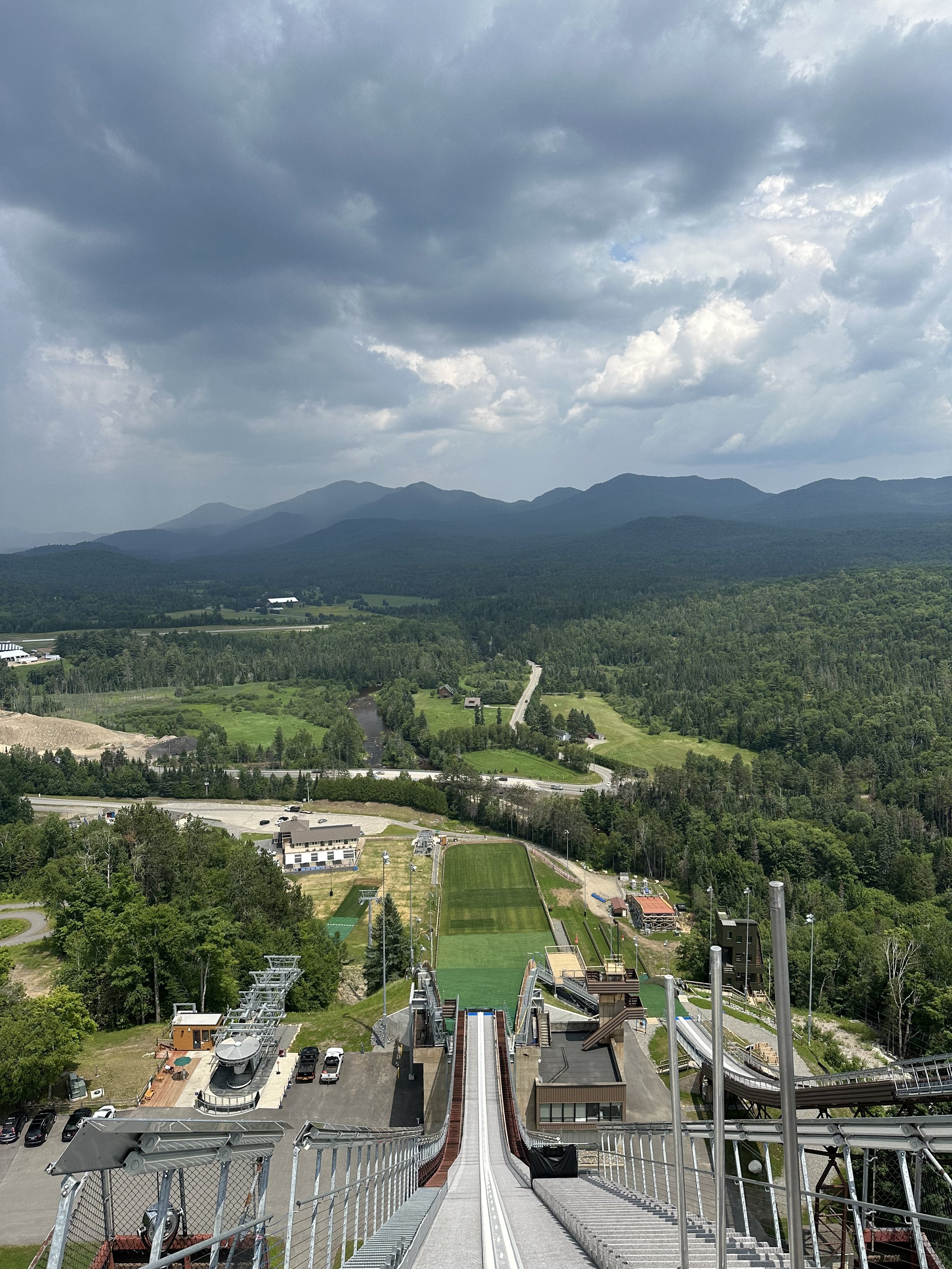The image captures a high-angle, aerial view from the top of a man-made ski jump set within a verdant, possibly mountainous region. The foreground features the ski ramp, flanked by fencing, descending steeply towards the ground. Off to the left, you can see a parking lot with a few cars and what appears to be a ski lift. The surrounding landscape is lush with green trees, indicating the season might be spring or summer. At the base of the ski jump, there are several small buildings and a green space shaped like a rounded rectangle. In the distance, additional buildings and highways are visible, set against a backdrop of dark blue mountains under a gray, cloudy sky that hints at imminent rain.